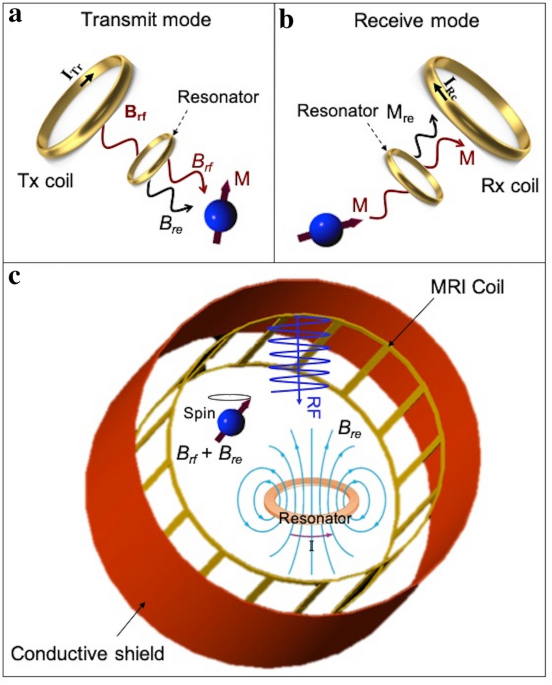The vertically aligned rectangular image consists of three sections labeled A, B, and C, each marked with a lowercase letter in the corner. Sections A and B, positioned side by side at the top, are smaller squares with white backgrounds and thin black borders. Section A is titled "Transit Mode" with a golden ring and coiled lines labeled "b sub re." A blue circle with an arrow and a capital M point to this structure. Section B, titled "Receive Mode," mirrors Section A but with coiled lines labeled "b sub rf" going in the opposite direction.

The larger square at the bottom, Section C, features a dominant red ring labeled "Conductive Shield" on the exterior, with an internal gold ring from which lines radiate in all directions. The center of this section is marked "Resonator." A blue ball labeled "Spin" appears in the upper left, with text "b sub rf + b sub re" beneath it. The upper right side of the gold ring contains the text "b sub re," and a coil with blue wavy lines and a down arrow labeled "rf" descends from the top. The exterior ring is marked "MRI coil" with an arrow pointing to the gold border. This detailed scientific illustration appears to visualize different operational modes and components of an MRI system, emphasizing the interaction between different coils, resonators, and magnetic fields.